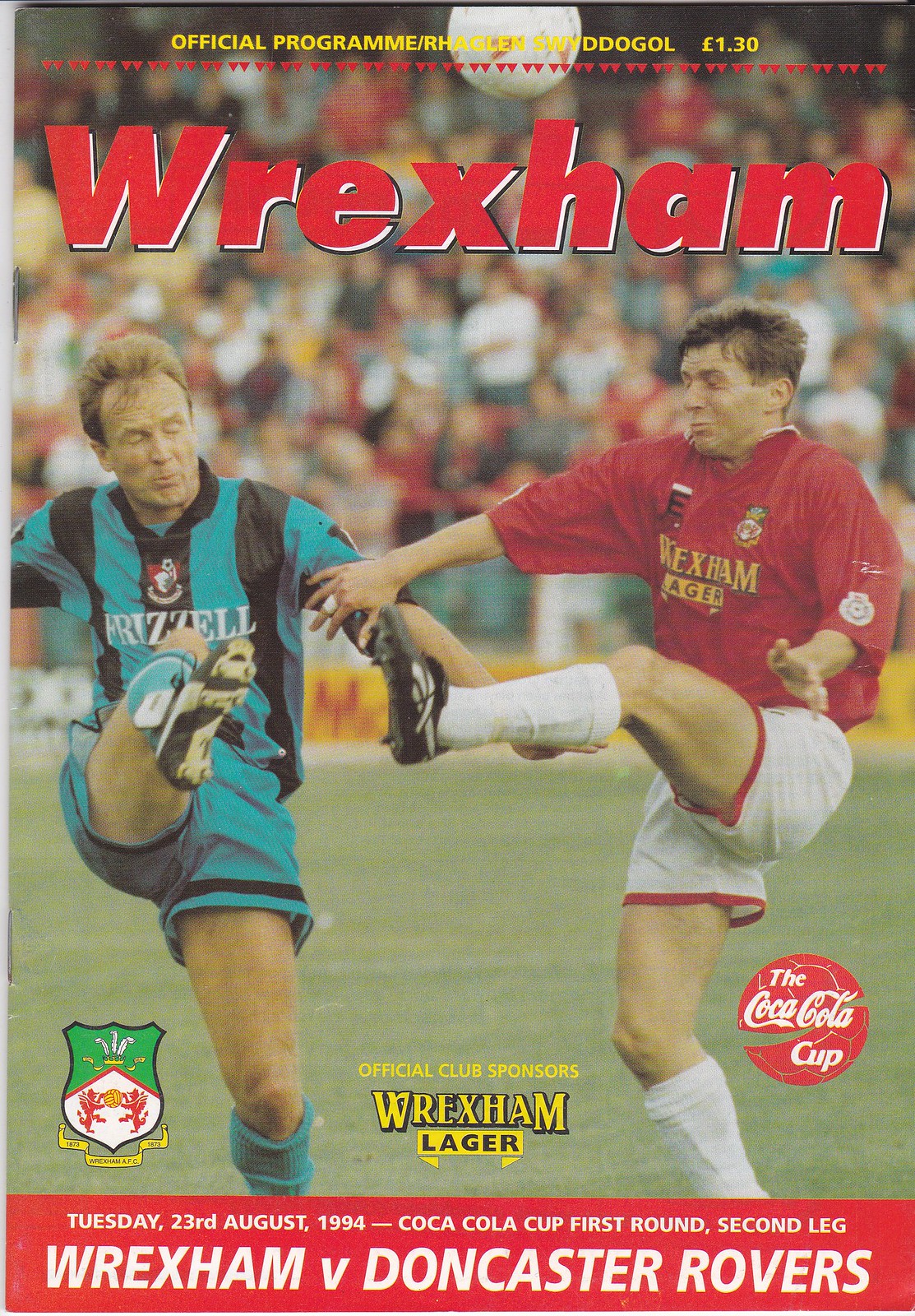The cover of the official Wrexham program is a vibrant and colorful image that predominantly features two players mid-action. The player on the right is in a red and white uniform, representing Wrexham, while the player on the left is in a blue and black striped uniform, likely from Doncaster Rovers. Both players have their eyes closed as they simultaneously attempt to kick a ball suspended in the air, giving the image a slightly amusing and dynamic appearance. 

At the top of the cover, "Wrexham" is boldly written in red, accompanied by the words "official program" in yellow. The cost is listed as 1.30 Euros. The bottom of the cover provides details about the match, noting it as taking place on Tuesday, 23rd August 1994, for the Coca-Cola Cup first round, second leg, between Wrexham and Doncaster Rovers. There is a red circle with a white inscription "Coca-Cola Cup" that resembles a soccer ball. Additionally, a logo featuring a green, white, and red shield appears on the left side with the text "Official Club Sponsors Wrexham Lager" in the center.